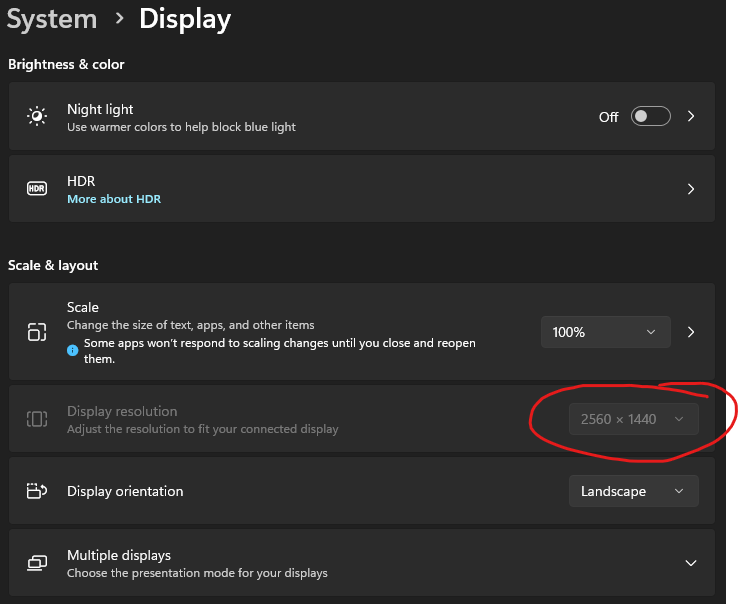The image depicts a screenshot taken from the system settings of a PC, set against a black background. In the upper left corner, the text "System Display" is prominently displayed in white, under which the section "Brightness and Color" is located. Just beneath this section, an icon resembling a light source is labeled "Night Light: Use warming colors to help block blue light," indicating that this feature is currently turned off.

Below it, the term "HDR" is present with a blue hyperlink stating "More about HDR." Moving further down, the section "Scale and Layout" is introduced. Beside this, there are several square icons; one labeled "Scale: Change the size of text, apps, and other items," which is currently set to 100%. A blue information icon notes that some apps won't respond to scaling changes.

Directly beneath is the "Display Resolution" section, advising users to "Adjust the resolution to fit your connected display." The resolution is set to 2560x1440, highlighted by a red circle to the right. Following this, the "Display Orientation" is marked as "Landscape" with an adjacent dropdown box for options.

The final section, "Multiple Displays," recommends users "Choose the presentation mode of your displays," accompanied by an icon of two small monitors on the left side of the title.